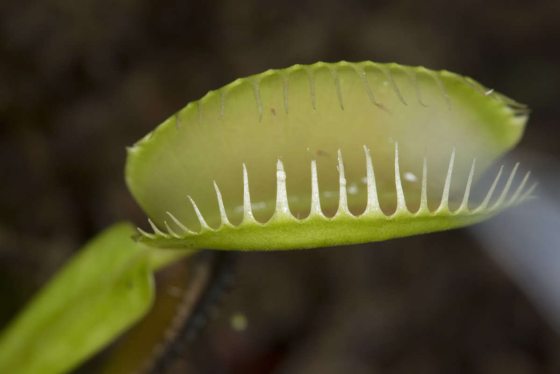This is an outdoor photograph showcasing a close-up view of a light green Venus flytrap at the center. The flytrap is open, revealing a lighter shade of green inside its "mouth," with distinctly white, spiky teeth lining the edges. The top half of the trap occupies the upper part of the image, while the bottom half is at the lower section. Adjacent to the flytrap, slightly below it to the left, there is a prominent green leaf, potentially another flytrap head facing a different direction. The blurred background consists of various shades of brown, possibly indicating soil or natural debris, with a mysterious white streak on the right side that could be caused by a light beam or something moving rapidly across the frame. The image provides a clear focus on the flytrap's details, emphasizing its readiness to catch an insect.